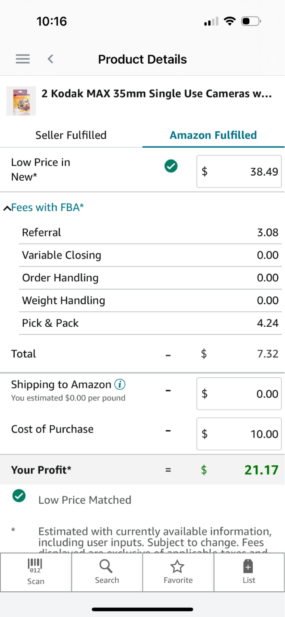This is a detailed description of an iPhone screenshot displaying product details from an Amazon seller tool:

---

The image is a screenshot from an iPhone, showing the product details page on a mobile application, likely an Amazon seller tool. 

- **Status Bar**: 
  - Top right corner: Two out of four signal strength bars are shown in light gray, with the connected bars indicated in black. Next to it are a black Wi-Fi symbol and a horizontally placed battery icon.
  - Top left corner: The time is displayed as "10:16" in black, against a light gray background.

- **Navigation Bar**:
  - On the left: A menu icon resembling a backward arrow (<) pointing to the left.
  - Center: The title "Product Details" in black, sans serif, title case letters. Below the title is a thin, one-pixel dark gray border line.

- **Product Section**:
  - An incomplete product title: "Kodak Max 35mm Single Use Cameras with..." indicates that its full name couldn't fit within the allotted space.
  - There are two sections for fulfillment options:
    - **Amazon Fulfilled**: Selected and highlighted in teal with a corresponding teal underline.
    - **Seller Fulfilled**: This option, in black letters, is not selected.

- **Amazon Fulfilled Details**:
  - **Low Price and New**:
    - This section has a green checkmark.
    - The price is listed as $38.49.
  - **Fees Breakdown**:
    - FBA fees: $7.32
      - Referral fee: $3.08
      - Variable closing fee: $0.00
      - Order handling fee: $0.00
      - Weight handling fee: $0.00
      - Pick and pack fee: $4.24
  - **Cost Breakdown**:
    - Price: $0.00
    - Cost of purchase: $10.00
  - **Profit Calculation**:
    - Displayed on a light gray background.
    - Profit: $21.17, shown in green with an asterisk.
  - **Additional Information**:
    - Green circle with a white checkmark stating "Low price matched."
    - A note mentioning estimations with current available information, subject to change fees, and user input.

- **User Interface Options**:
  - At the bottom of the screen, there are four navigation buttons: "Scan," "Search," "Favorite," and "List."

---

This caption provides a comprehensive and detailed description of the screenshot, capturing the essential elements visible on the iPhone's screen.